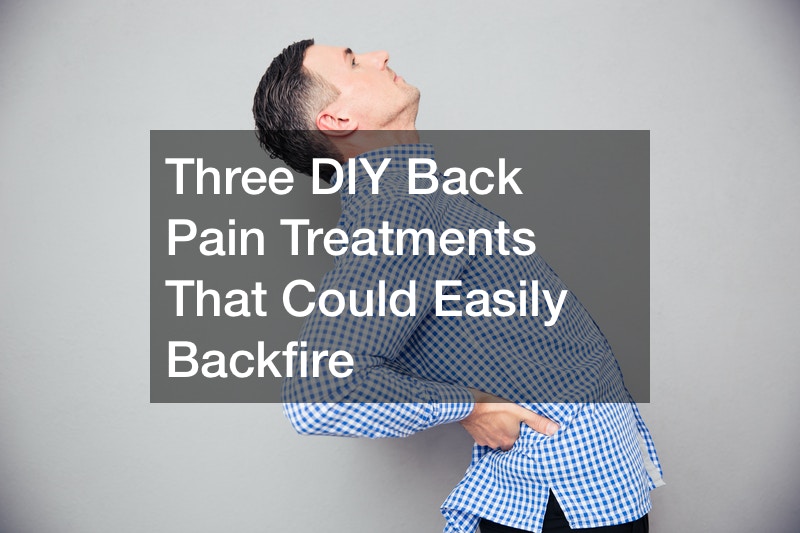This image resembles a cover page or poster typically seen in a medical setting, possibly a doctor's office. At the forefront is a man wearing a blue and white checkered shirt and black pants, captured from the waist up. He is leaning backwards with his hands on his hips or lower back, indicating discomfort. His expression is one of pain, and he is looking upward at a 45-degree angle. The background is light gray, which contrasts with an opaque gray text box centrally located in the image. This text box contains the white-lettered title: "Three DIY Back Pain Treatments That Could Easily Backfire." The arrangement of the text is on four lines, ensuring it stands out prominently against the subdued background. The overall composition effectively conveys the theme of back pain treatments gone wrong, highlighting a man in visible discomfort.